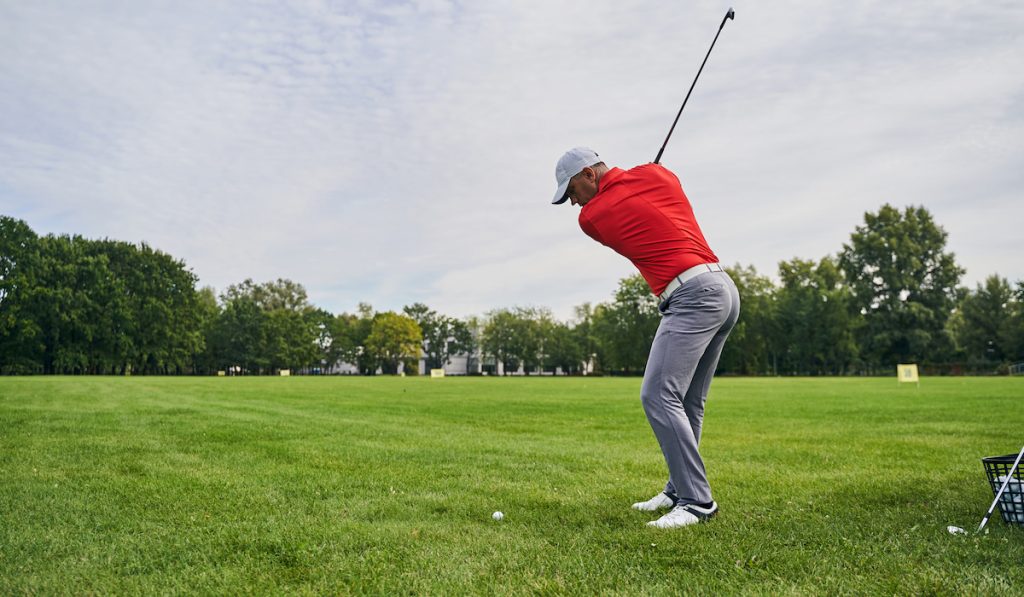This vibrant color photograph captures a male golfer mid-swing on a sprawling, green golf course. The golfer, dressed in a red polo shirt, gray pants with a white belt, and white and black shoes, is also sporting a white cap. He stands slightly right of center, eyes focused on a white golf ball resting on the neatly manicured grass. His golf club, raised high behind him, indicates that he is about to take his shot. 

In the foreground to the right, a black plastic basket filled with additional golf balls can be seen beside another golf club leaning against it. The expansive, flat golf course extends behind him, bordered by a row of lush green trees that suggest a summer or spring setting. On the horizon, white buildings, possibly a clubhouse, are visible. A prominent yellow sign is also discernible among the buildings. The daytime sky above is a blend of blue and scattered clouds, adding to the serene and focused atmosphere of the scene.